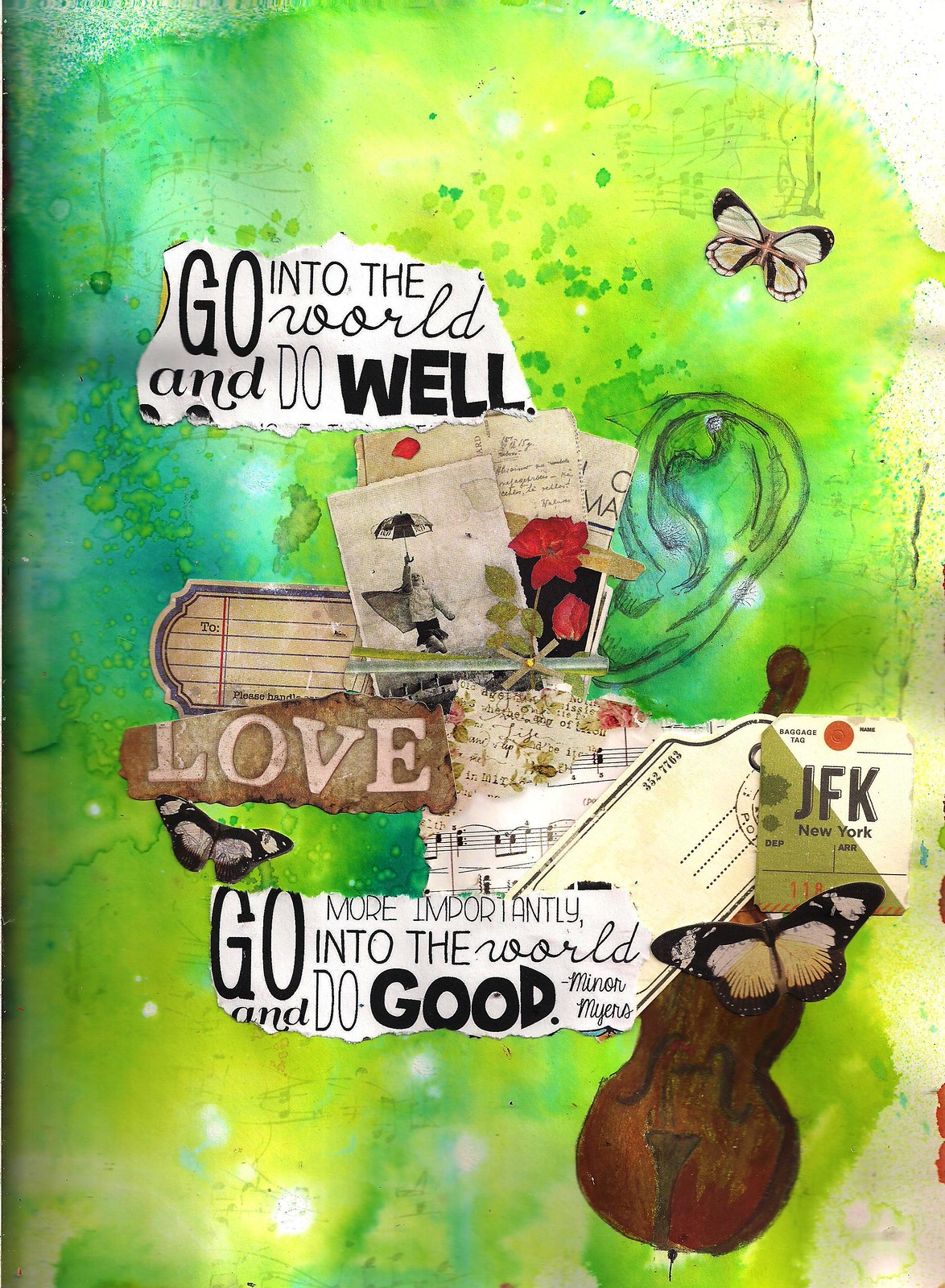The image is a detailed and vibrant collage featuring a variety of elements layered over a bright background splattered in shades of lime green, yellow, and hints of aqua blue. At the center of the composition, amidst the chaos of details, several key elements stand out:

1. **Drawings and Images**:
   - A prominent drawing of an ear catches the eye.
   - Multiple butterflies are scattered across the collage, with one notably positioned in the upper right corner.
   - A photograph of a flower adds a touch of natural beauty.

2. **Textual Elements**:
   - Two inspiring quotes are pasted separately: "Go into the world and do well" located on the upper left, and "Go more importantly into the world and do good. Minor Myers" integrated into the lower part of the image.
   - The word "LOVE" is torn out from another piece of paper and prominently displayed.

3. **Musical and Postcard Motifs**:
   - Torn sheet music is featured, contributing to the theme of art and creativity.
   - An image of a cello is placed towards the bottom, enhancing the musical motif.
   - A facsimile of a ticket marked "JFK New York" evokes a sense of travel and adventure.
   - Postcards and additional fragments of handwritten notes add to the nostalgic and eclectic feel.

This intricate montage creates a rich tapestry of visual and textual elements, blending art, music, and inspirational messages to craft an evocative and multilayered artwork.